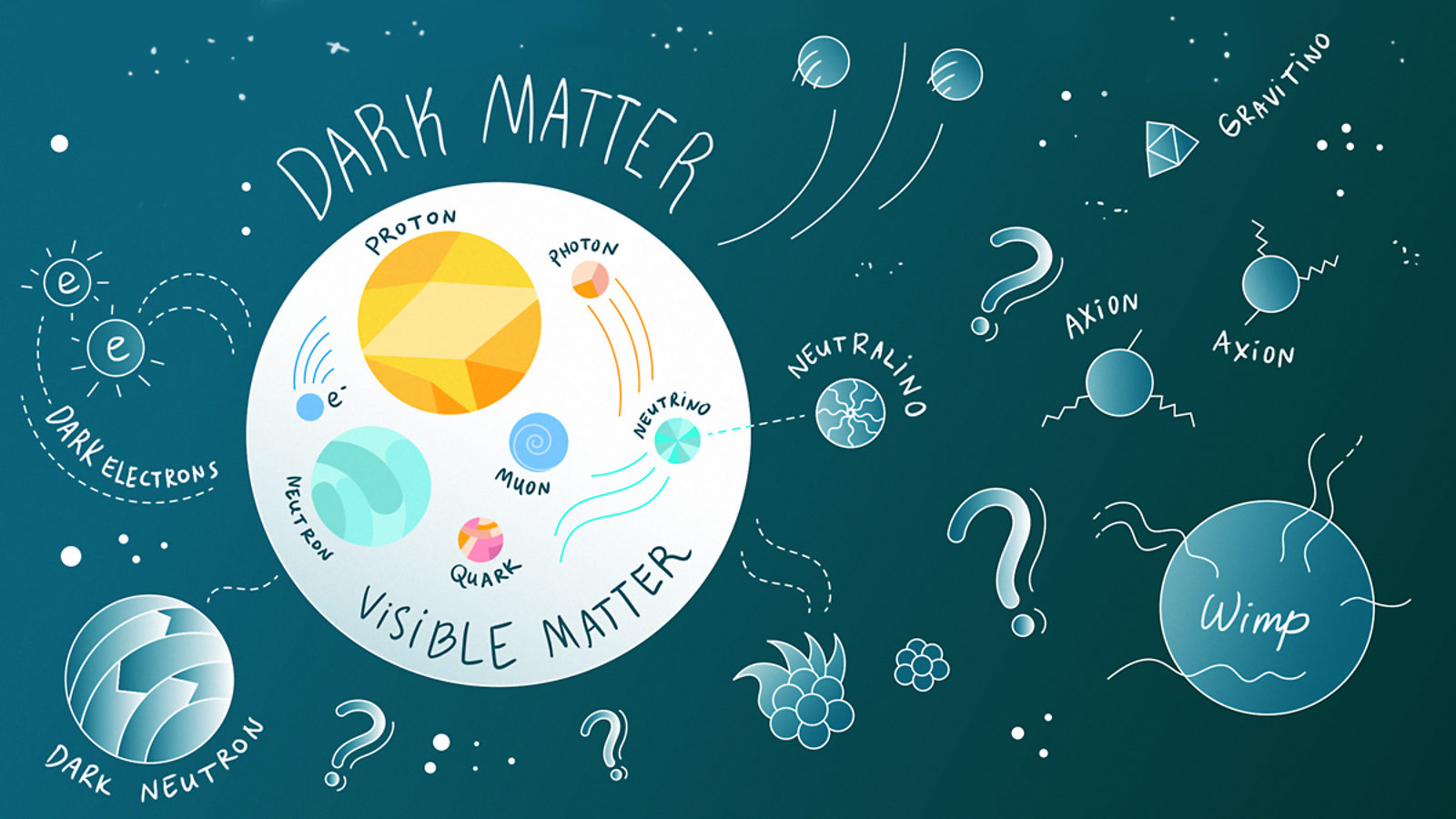This image is a detailed and comprehensive poster designed to explain dark matter and visible matter, likely aimed at students or young people. The background is a dark teal, resembling the night sky. Central to the poster is a prominent white circle labeled "visible matter," containing colorful depictions of various subatomic particles such as protons, neutrons, photons, muons, neutrinos, quarks, and electrons, all marked with different colors like yellow, teal, blue, pink, peach, and orange. These particles are interconnected with lines, highlighting their interactions.

Surrounding this white circle is a larger dark blue area representing "dark matter." It includes illustrated elements like dark neutrons, dark electrons, gravitinos, axions, and neutrinos, depicted with swirly and dotted lines, along with question marks that suggest the mysterious nature of these particles. Notably, in the lower right corner, there’s a big circle labeled "WIMP" with swirling lines converging into it.

The poster is visually compelling with hand-written styled fonts and animated elements to engage young viewers, helping them understand the difference between visible matter and the more enigmatic dark matter.